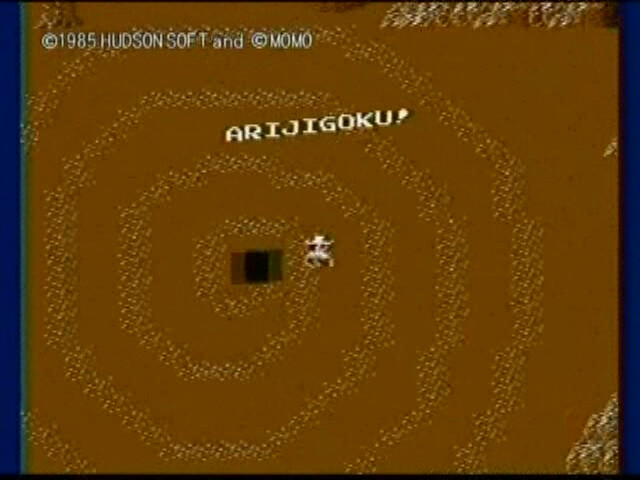This detailed screenshot from a classic video game, possibly from the 1980s, features a captivating visual layout. Encased in a blue border, the main part of the image is dominated by a textured brown background accented with lighter brown swirls, giving it a granulated appearance. At the center of these swirling patterns lies a prominent black square. To the right of this square, there is an enigmatic white figure that might resemble an animal or another entity, adding an element of mystery to the scene. The top of the image is marked with the bold text "ARIJIGOKU!" while the top left corner credits "1985 Hudson Soft and Momo," anchoring the screenshot firmly in its retro origin.